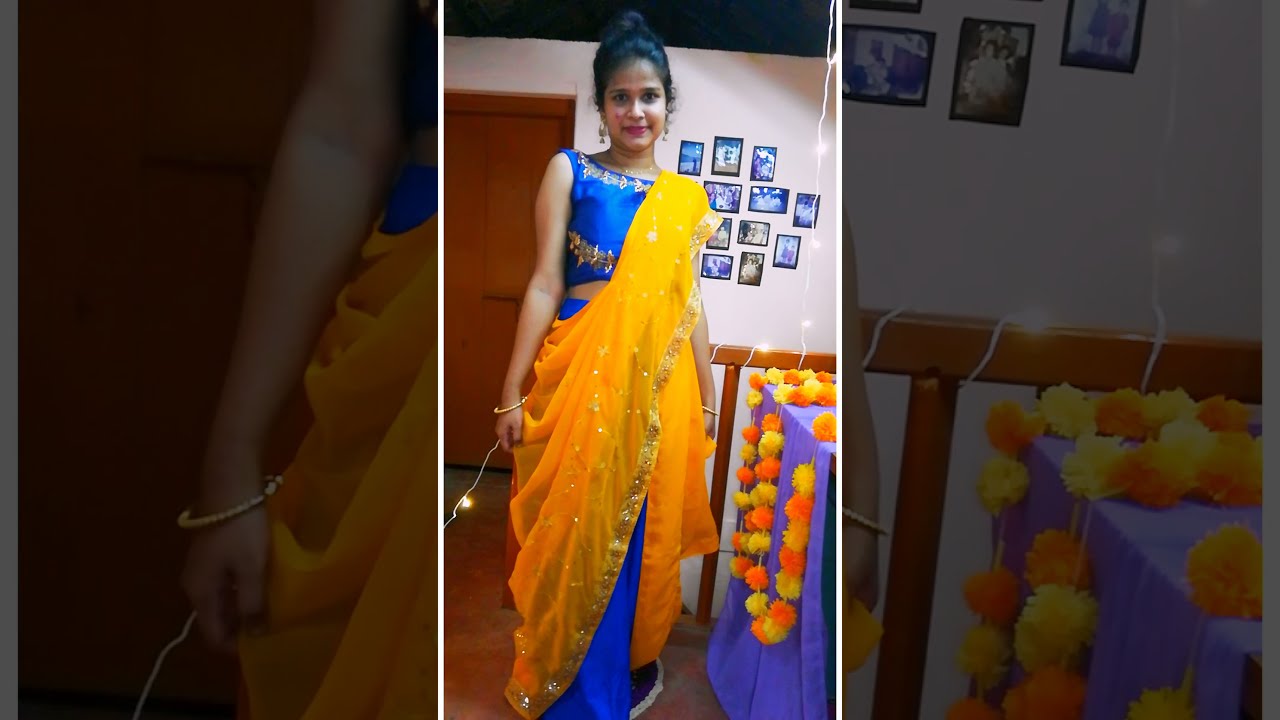The image depicts a young Indian woman wearing an ornate Hindu-style dress, often referred to as a sari. The dress features a sleeveless, blue top section with intricate ornamental lines and gold applique inlay. A matching blue skirt extends to her ankles. Adding to the elegance, a flowing yellow sash adorned with white stones and shiny crystals drapes from her left shoulder down to her right hip, reaching the floor. The woman’s hair is styled up, and she is accessorized with dangly earrings, emphasizing her made-up appearance.

The scene is set indoors, where the woman stands next to a platform draped in purple fabric. Hanging from the platform are large, puffy necklaces comprised of alternating orange and yellow puff balls, resembling marigold strands or leis. Behind her, an off-white wall is adorned with a few framed pictures, creating a homely ambiance. This detailed backdrop not only highlights the intricate details of her attire but also suggests she might be preparing for a cultural event or celebration. The central image is vertically framed, with an identical picture zoomed in and faded out as the background, further emphasizing her traditional and beautiful appearance.